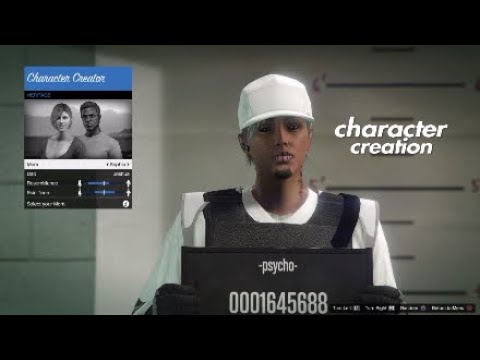In this image, the main focus is on a user interface from a character creation tool. At the top and bottom of the frame are black boxes, possibly part of the interface's design. The background is gray, resembling the facade of a house. 

At the center, there's a person wearing a black vest over a white shirt and a white cap, possibly the character being created. To the left of this character is a small box with a blue header that reads "Character Creator" in white text. 

This box features a gray background showcasing two characters, a man, and a woman. Just below this image is a white line followed by another black box containing some white text, two small blue lines, and some upward-pointing white arrows, likely interface elements for character customization.

At the bottom-left of the character, there is a black box displaying the text "psycho 0001645688" in white. To the right of this box, the words "Character Creation" are printed in white text. 

In the background, a measuring wall is visible with markings at six feet, five feet, and other intervals, possibly indicating the character's height. Finally, the bottom of the image contains very small, white print.